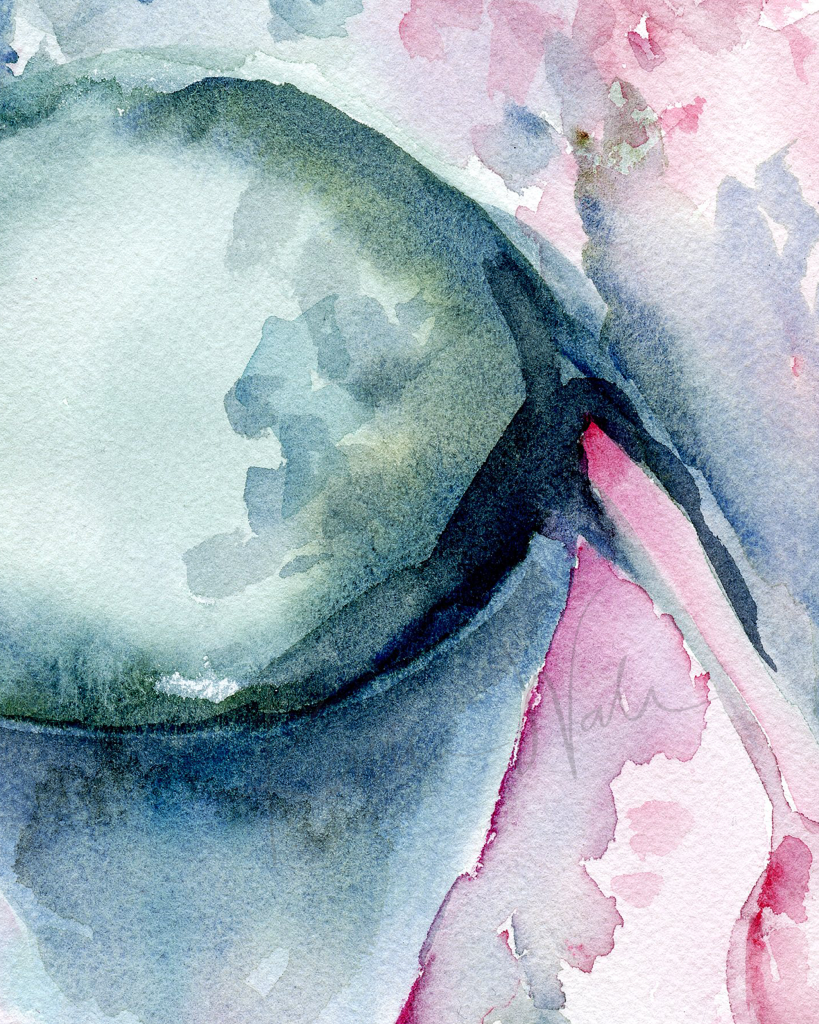This detailed abstract watercolor painting predominantly features hues of blue, aqua green, and pink. The image is characterized by fluid paintbrush strokes that bleed and blend into each other, exemplifying the typical attributes of watercolor art. The painting showcases a balance between darker and lighter elements, with deeper navy blue and dark green tones melding into lighter mint green, aqua, and soft pink shades. 

The composition is somewhat split into two portions: the left side mainly displays the aqua and blue areas, particularly forming an egg-like shape in the middle. Within this shape, the aqua lightens towards the left edge and becomes a darker shade as it approaches the pink on the right. The pink areas are mostly located on the lower and upper right portions of the painting and are interspersed with blue flecks and white blotches, creating a textured burst effect. 

There's an intriguing section where aqua green and blue 'fingers' leap into the pink towards the middle, adding complexity to the interplay between the colors. The texture and layers are built up through visible brush strokes, adding depth to the abstract composition. Though the painting may initially appear difficult to decipher, some interpretations suggest a conceptualized form suggestive of anatomical shapes like a uterus, although this remains open to interpretation.

The piece bears the artist's signature, potentially reading 'Vala' or 'Vara,' written with a purple hue more prominently visible on the right side.